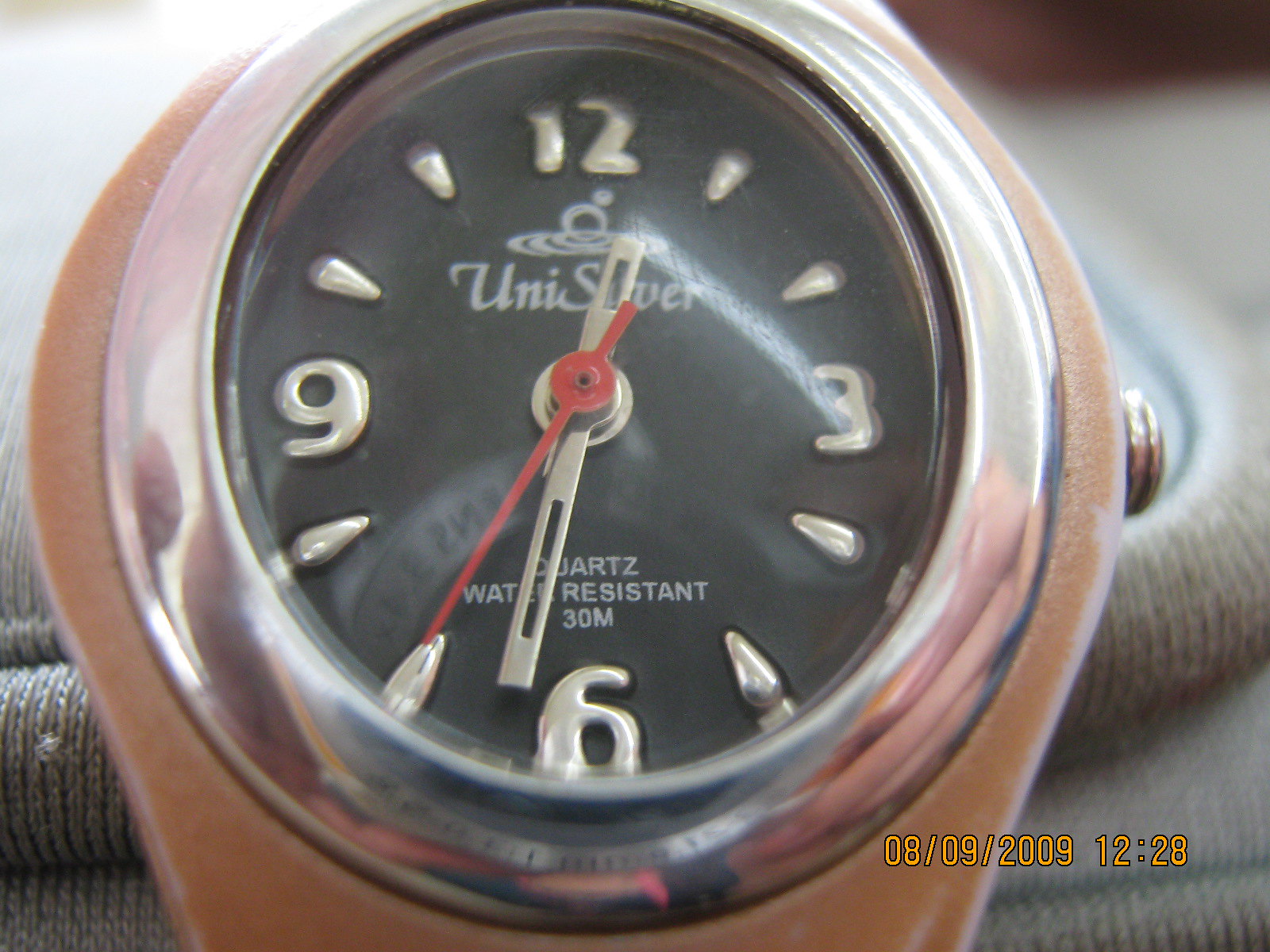This is an intricately detailed close-up photograph of a wristwatch face. The scene captures the watch at 12:28 PM, as indicated by the bright yellow, slightly orange timestamp located in the bottom right of the image. The date imprinted is August 9th, 2009. The ambient lighting in the photo suggests that it was taken during daylight hours due to the brightness and quality of the light. 

The watch, identified as a Unisilver Quartz model, boasts a water resistance capability of up to 30 meters. The watch face itself features a sleek black background, drawing a stark contrast to the silver-painted numerical hour markers. Both the minute and hour hands are also silver, harmonizing with the numerics, while the second hand stands out in a vivid red. The entire composition emphasizes the sophisticated design and functionality of the timepiece.